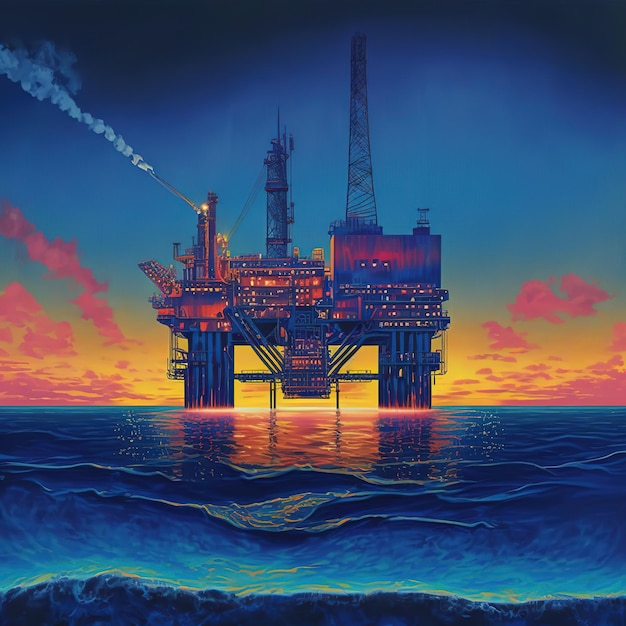This digital illustration captures a vivid, computer-generated image of an oil rig majestically standing in the middle of a rippling ocean. The dramatic sky transitions from a royal blue at the zenith to a fiery orange and yellow at the horizon, suggesting a stunning sunset or sunrise. Pink clouds are streaked across the sky, enhancing the vibrant palette. The central focus is the metal oil rig, which is elevated on two substantial pylons. It includes various features such as towers, antennas, lights, and a smokestack emitting white smoke. The ocean reflects the sunset’s hues with its surface displaying a mesmerizing interplay of dark and light blues, highlighted by yellow and orange-pink accents. The combination of colors and elements creates a surreal, almost cartoonish yet lifelike scene.